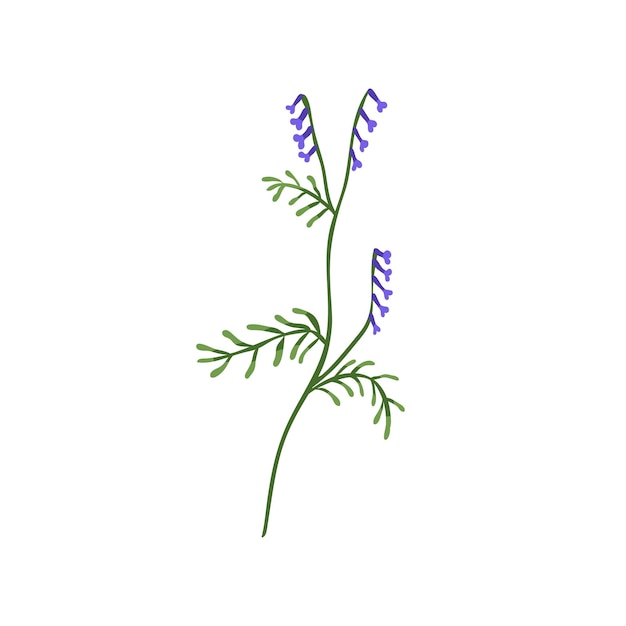This is a vertically oriented drawing featuring a gracefully curved green stem with several branches extending outward, set against a stark white background. The lush green stem originates from the bottom left, curving gently as it ascends and splits into multiple branches. Towards the top, the stem forms a V shape, with both arms of the V adorned with bluish-purple, bell-shaped flowers. There are about four blooms on each of these upper branches. Additionally, a lower branch on the right also showcases five similar flowers. The flowers are elegantly fluted, resembling small bells, contributing to the delicate appearance of the image. Interspersed among the flowers are thin, dark green leaves with lighter green tips, further enhancing the organic feel of the illustration. The overall simplicity and clean lines suggest that the image might be a hand-drawn or digital sketch, focused solely on the botanical elements with no text present.